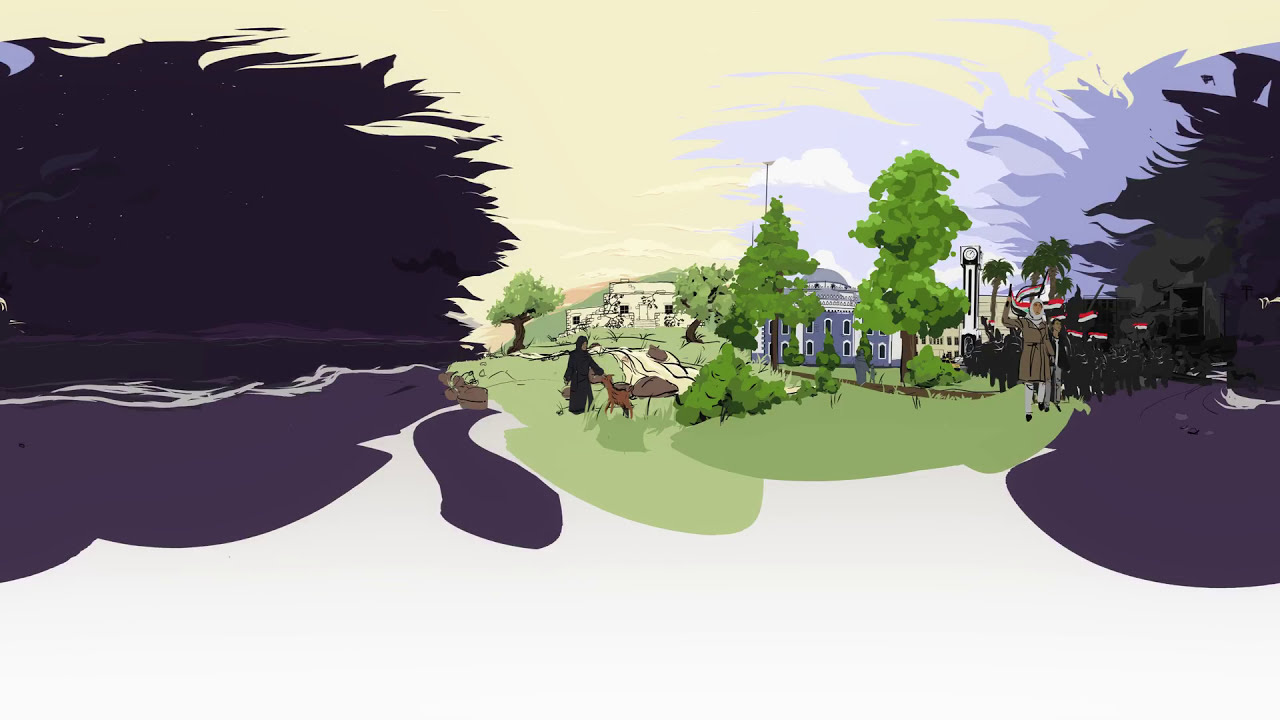The image is an illustration depicting a contrasting and surreal scene. In the center, there's an oasis-like area with green grass and trees under a yellow and blue sky, providing a stark contrast to the darker surroundings. A woman wearing a hijab is seen tending to or petting a goat. Nearby, another woman, dressed in black from head to toe, is accompanied by a small brown dog. The middle part of the image showcases an administration building with a dome, surrounded by people walking around.

On both the left and right sides of the image, the sky is dark blue with hints of purple, creating a mysterious and almost ominous atmosphere. The left side features what appears to be rough waters or an abstract storm-like scene with shadowy and grey areas. To the right, there's a group of people carrying flags with red, white, and black stripes, which suggests a protest or march. In the background, there are additional buildings, with one being green and another dark grey, partially obscured by trees. This rich and detailed illustration leaves an intriguing mix of political, natural, and surreal elements.